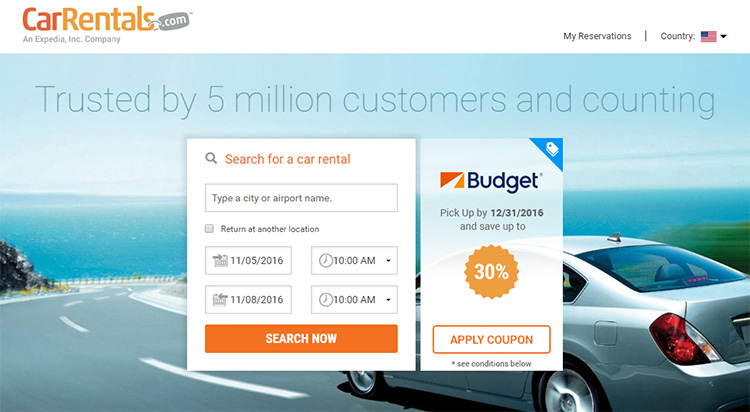The screenshot showcases the homepage of CarRentals.com, an online platform for booking car rentals. The logo is prominent in the upper left-hand corner, where "Car" is depicted in red, "Rentals" is in a yellowish-orange hue, and ".com" is written in white on a gray keychain. The website operates under the umbrella of Expedia Inc., noted at the top of the screen.

In the top right section, users can access "My Reservations" and select a country from a dropdown menu, with the United States currently selected. The central focus of the image features a picturesque silver car driving along a road marked by white lines, indicative of one-way traffic, although this detail might be inaccurate. The car is on a scenic, winding route adjacent to a hillside that offers sublime views of a vibrant blue ocean, suggesting the landscape is likely the West Coast of North America, possibly California.

A tagline on the site reads, "Trusted by 5 million customers and counting," in a subtle, dark, thin font. Below this, users can see two interactive sections. The first is for searching car rentals, where one can input the city or airport, choose if returning to a different location, and specify the pickup and return dates and times. A prominent orange "Search Now" button facilitates the search.

Beneath the search section, there's a promotional offer for Budget car rentals. Users are informed they can save up to 30% if they pick up their rental by December 31, 2016. The promotion highlights an option to apply a coupon code for additional savings.